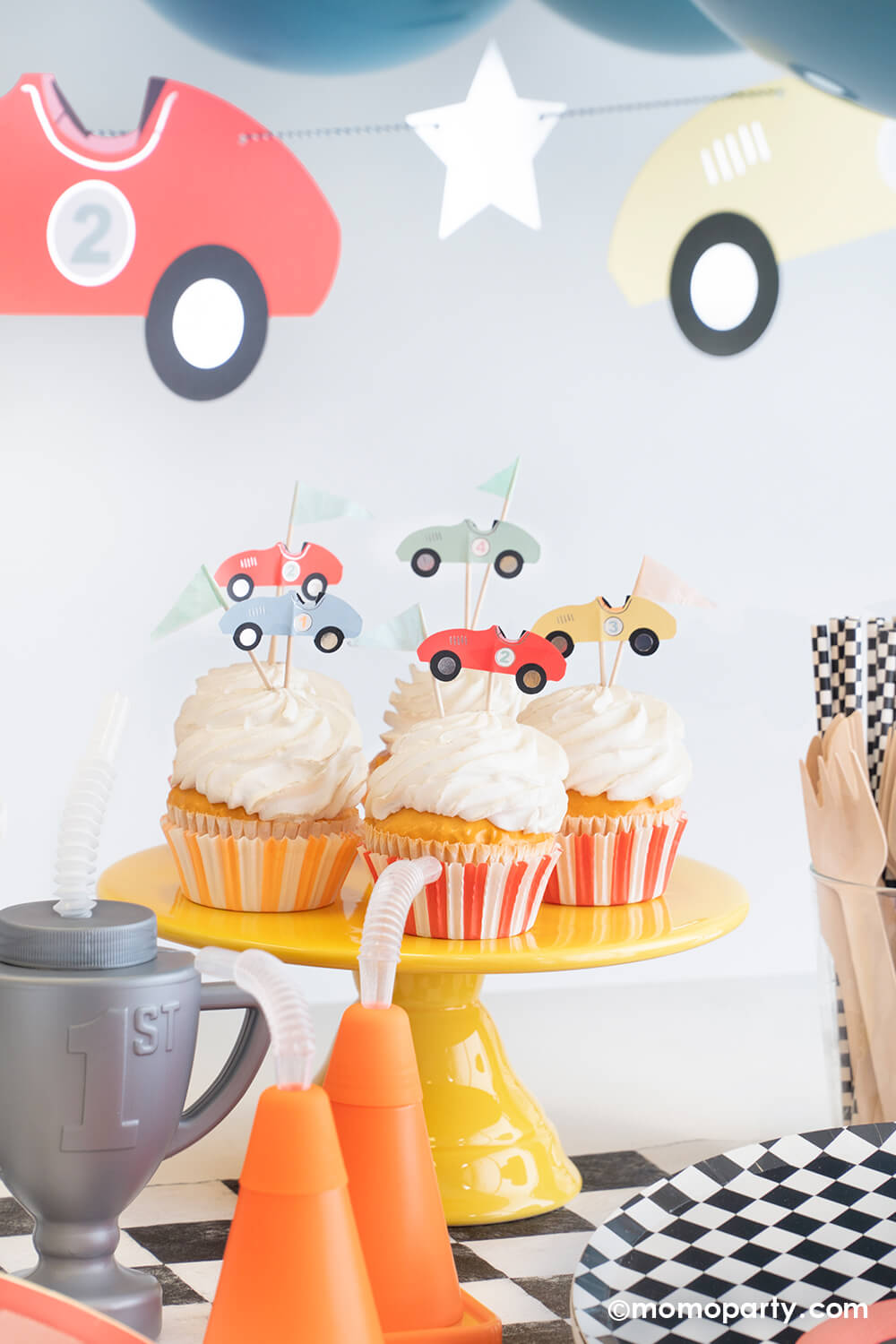This vivid photo captures a lively, race car-themed birthday party scene set inside what appears to be an ice cream parlor or dessert shop. Dominating the scene is a bright, shiny yellow ceramic cake stand showcasing five giant cupcakes, each adorned with white whipped cream frosting. The cupcakes are nestled in striped cupcake wrappers of red and white or yellow and white, and are topped with miniature race car decorations in red, blue, yellow, and turquoise. Accompanying each race car is a small pennant flag in turquoise, blue, and pink, all held by toothpicks.

In the background, the wall features painted race cars and stars, enhancing the theme. The table in the foreground is covered with checkered flag-patterned items including plates, drinking straws, and napkins rolled in a vase. To the right, there is another checkerboard-patterned table displaying additional thematically consistent decorations, such as traffic cones and a gray trophy labeled "FIRST". The festive atmosphere is completed with red and yellow birthday banners shaped like race cars, adding a dynamic and celebratory feel to the scene.